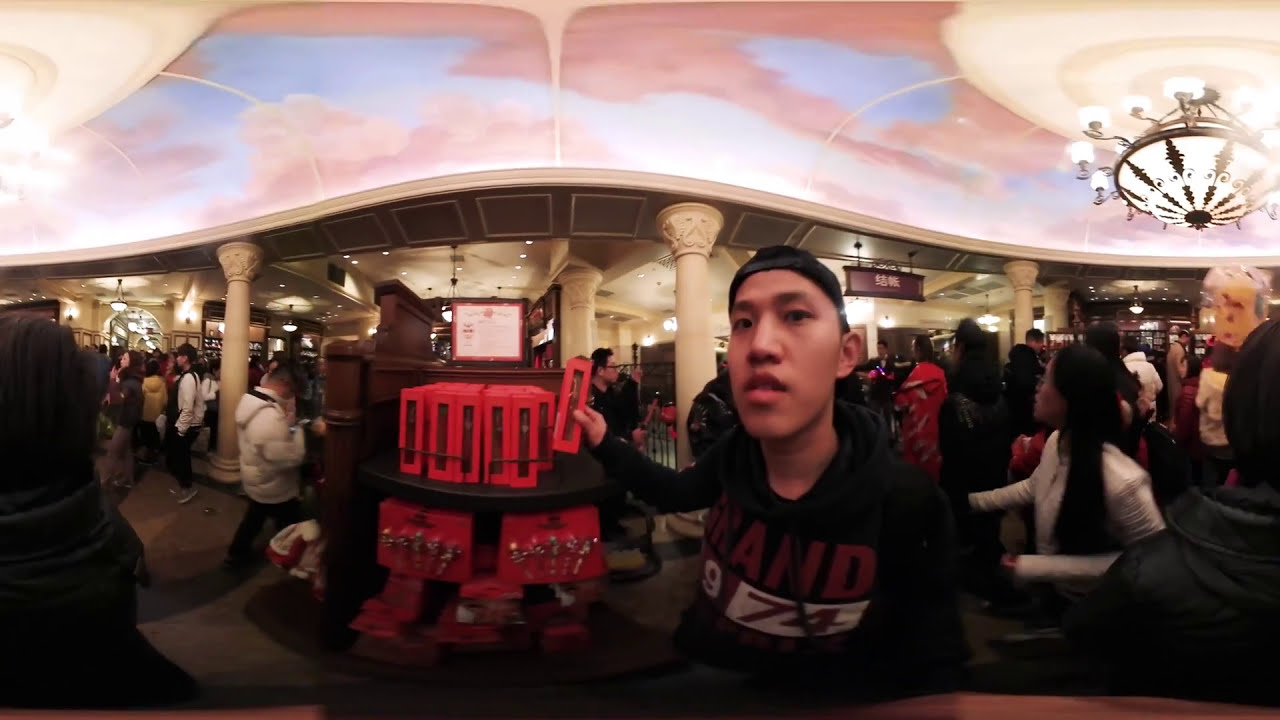In the photograph, a young Asian male, likely in his college years, occupies the foreground. He wears a black baseball cap turned backward and a black long-sleeve sweatshirt featuring red letters "AD," a white number "9," and the numbers "74" in red, set against contrasting red and white boxes. The man appears to be picking up a red-boxed item from a brown shelf laden with identical packages, possibly souvenirs. He is holding the object in his right hand, poised as if examining it. The bustling background reveals a crowded indoor space resembling a shopping mall or casino, with numerous people engaged in various activities. The ceiling is artistically painted to resemble a blue sky marbled with pink clouds, complemented by elaborate white and gold chandeliers. Large columns also punctuate the space, which adds to the grandeur of the setting. The atmosphere is lively, with people scattered throughout, some standing near slot machines, indicating this vibrant environment might be a casino or a busy commercial area.